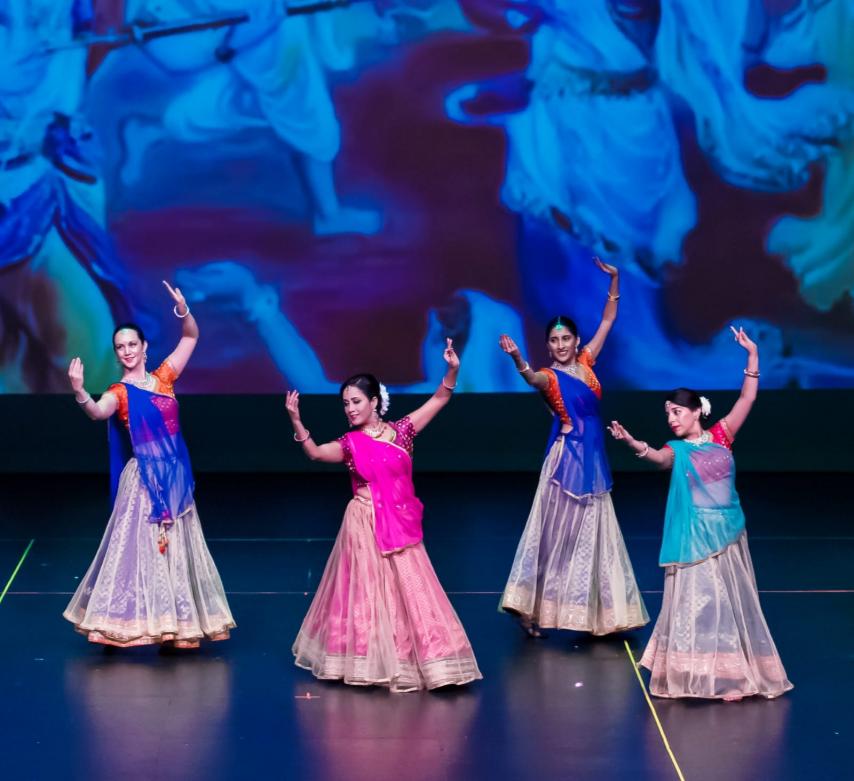This color photograph captures a vivid and dynamic performance of four East Asian women dancing on a dark, shiny stage. They are dressed in traditional Indian attire, each adorned in brightly colored blouses and matching long, flowing skirts with sheer overlays that reach the floor, concealing their feet. The women are positioned two in front and two behind, all with their arms raised identically above their heads, left arm slightly higher than the right, and gazing off to the left in unison.

Their hair is dark, parted down the center, and pulled back, adorned with either bright forehead marks or jeweled headpieces, some featuring flowers. Each dancer wears wrist bangles and unique color combinations: one in light blue, one in pink, one in dark blue, and the last in another shade of blue. The light illuminates their vibrant clothing against a backdrop characterized by blue and darker blue shades, possibly featuring abstract shapes or additional dancer images, creating a mesmerizing scene that enhances the overall theatrical experience.